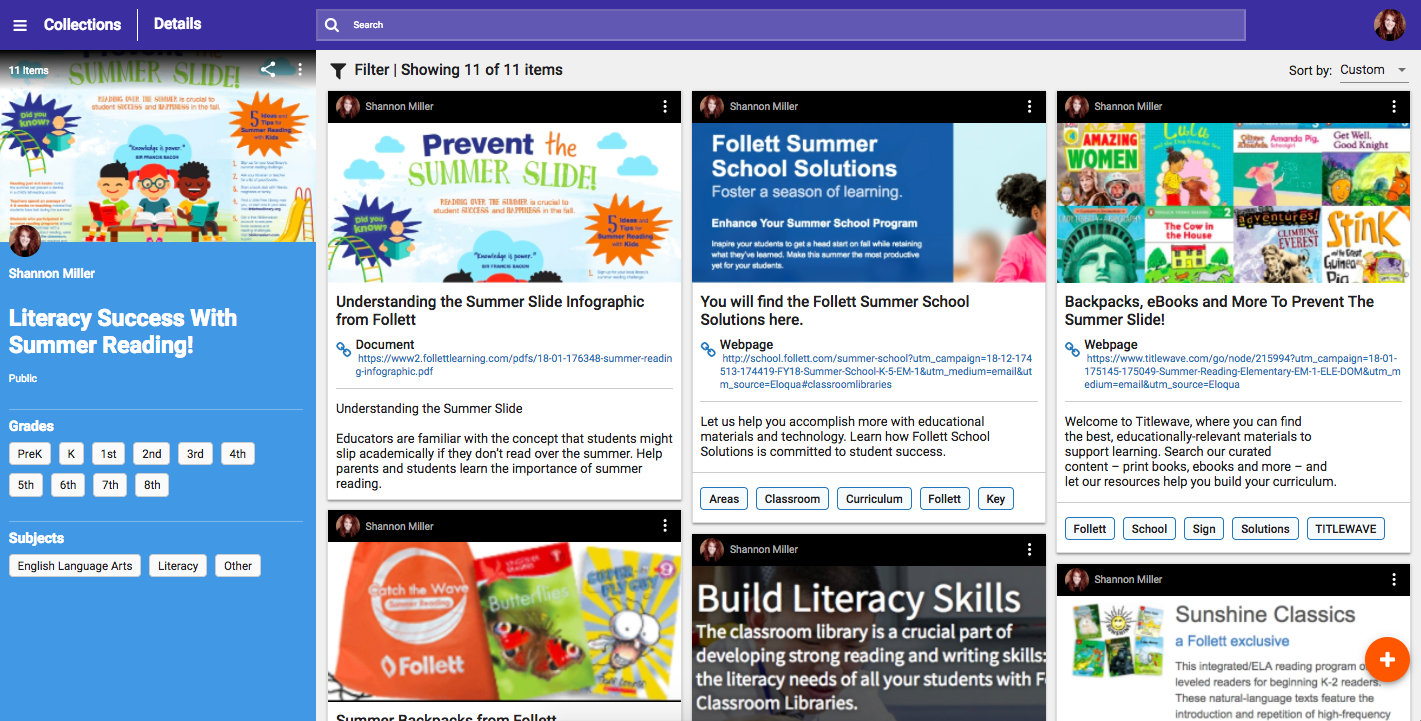This is a detailed screenshot of a website interface. At the top left corner, there is a rectangular purple button featuring three horizontal lines, likely indicating a menu that can be expanded. Adjacent to this button, in white font, are the words "Collections," followed by a small white vertical line, and then the word "Details." 

Next to this section is a long rectangular search field with a white magnifying glass icon on the left side. The placeholder text "Search" is displayed within the search bar in white font. On the upper right side of the header, there is a profile picture depicting a Caucasian woman with brunette hair, showing only her head.

Below this header section, the main content of the webpage is visible. Here, there are two horizontal rows, each containing three suggested articles personalized for the user. Each article preview is topped with a black banner displaying the name "Shannon Miller." 

The first article in the top row is titled "Understanding the Summer Slide Infographic from Follett." The second article in this row is titled "You'll Find the Follett Summer School Solutions Here." Each article appears to be tailored to Shannon Miller's interests and recommendations.